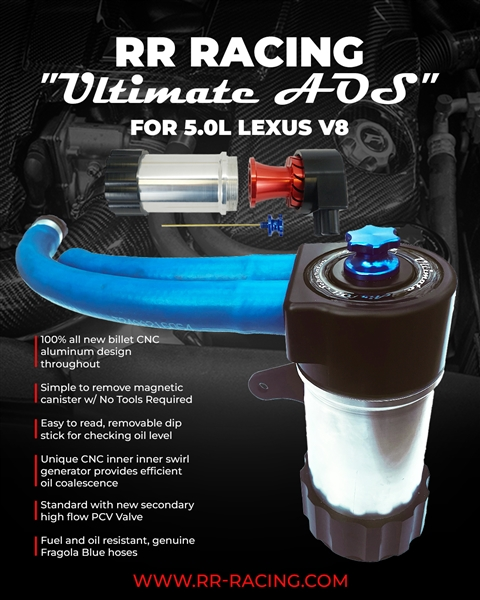The advertisement showcases a sophisticated racing engine part designed specifically for 5.0L Lexus V8 engines, prominently labeled as the "RR Racing Ultimate AOS." The backdrop is predominantly black, creating a striking contrast with the detailed imaging and informative text. The focal point is a cylindrical component featuring a grey base, a black top, and distinctive blue elements including tubes and a knob. A car engine is subtly visible in the background, reinforcing the automotive context.

Accompanying the image is white text at the top declaring "RR Racing Ultimate AOS" for the specified engine type. Detailed bullet points on the left outline the part’s features, such as a tool-free, magnetic canister removal, an easy-read, removable dipstick for oil level checking, and numerous advanced attributes like a 100% all-new billet CNC aluminum design and fuel-resistant Fragola hoses.

At the bottom of the advertisement, a series of six red vertical lines divides additional features, emphasizing the product's engineering precision and user-friendly aspects. The ad also includes the company’s website, www.rrracing.com, highlighted in red text, providing a direct link for further information or purchase.